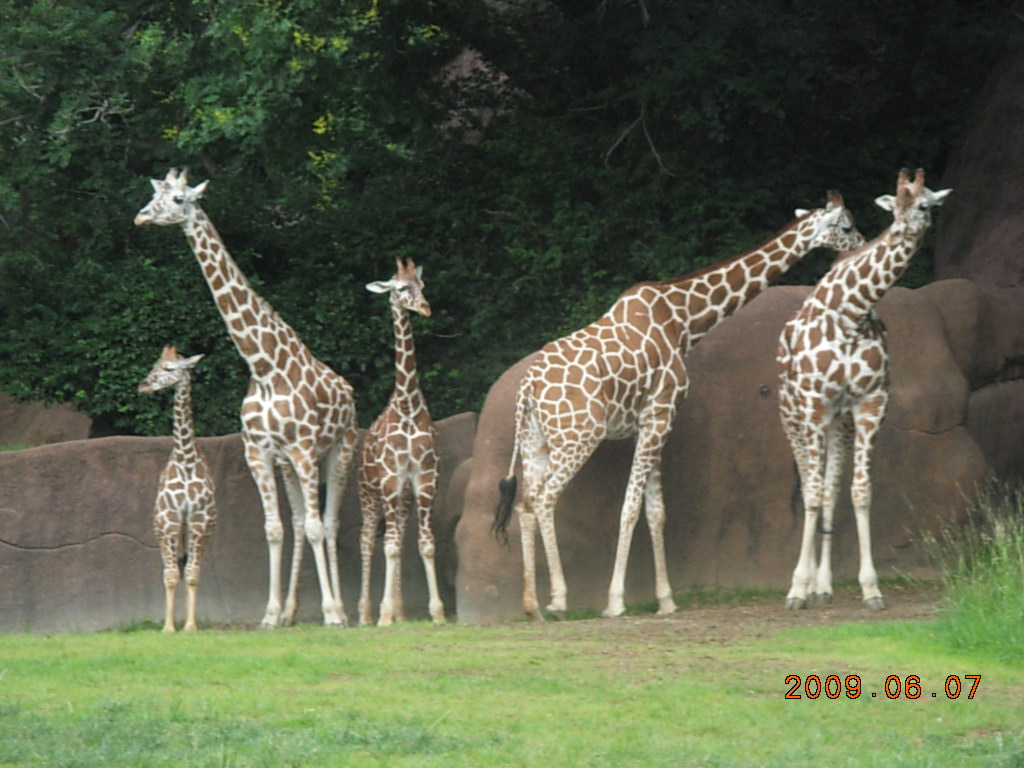This color photograph, dated June 7th, 2009, captures a group of five giraffes at a zoological park. The giraffes are standing in an enclosure, though the walls and fences are not visible in the image. The foreground features a mix of grass and bare dirt, likely trampled by the animals, with a tall clump of grass on the lower right. In the background, artificial brown boulders, likely made of concrete, span the width of the photo, blending with a wall of greenery and tree limbs arching into the frame from the top.

Among the giraffes, there are three adults and two young ones. The smallest giraffe, a calf, stands on the far left next to an adult whose neck is tilted to the side, with its head facing left. The middle giraffe, slightly taller and possibly a teenager, holds its neck straight up with its head angled slightly to the right. Another adult stands to the right, shown in profile as it appears to be walking towards the right edge of the photo. The last adult giraffe faces the camera directly, with its neck bent at an unusual angle, possibly resting its head on its back. The photograph is date-stamped in red font in the lower right corner, marking the day as June 7th, 2009.